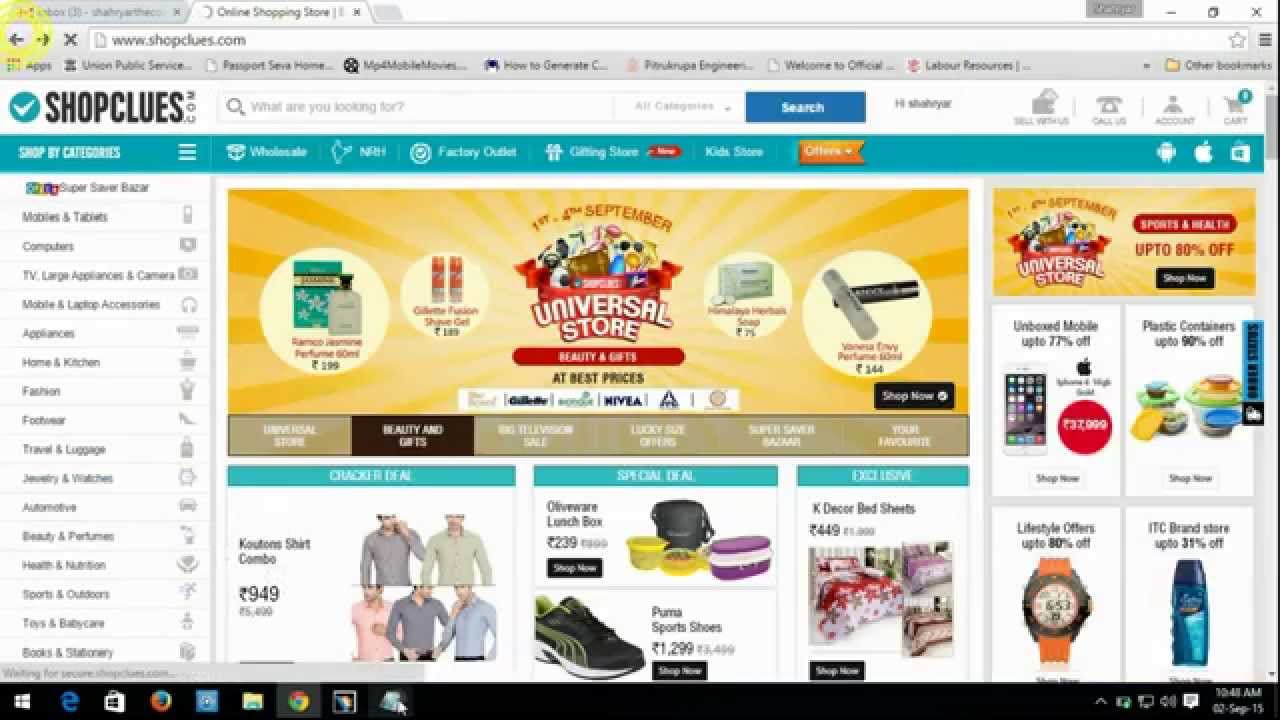Screenshot of a ShopClues.com Shopping Page

This screenshot captures the main interface of the ShopClues.com shopping page. The header features the ShopClues logo—a turquoise circle with a white checkmark, followed by the site name "ShopClues.com" in black text. To the right of the logo is a search bar where users can type their desired items, accompanied by a drop-down menu set to "All Categories." A blue search button with white letters is positioned next to the search bar.

On the same line, the page greets the user with a "Hi" followed by a blurred-out username, ensuring privacy. Adjacent to this are icons representing a phone, an account, and a shopping basket that already contains one item.

Below the header is a turquoise banner with white text that reads "Shop by Categories." Following this banner, a navigation menu includes tabs for "Factory Outlet," "Gifting," "Crafting Store," "Kids Store," and "Offers," the last of which is highlighted with an orange light banner. There is also an option for "Wholesale."

Under the "Shop by Categories" section, several categories are listed, including "Mobile Tablets," "Computers," "Large Appliances," "Cameras," "Fashion," and "Footwear."

The central area of the page displays advertisements for products available on the site, showcasing items such as shirts, shoes, lunchbox Tupperware, an Apple tablet, a watch, and other containers.